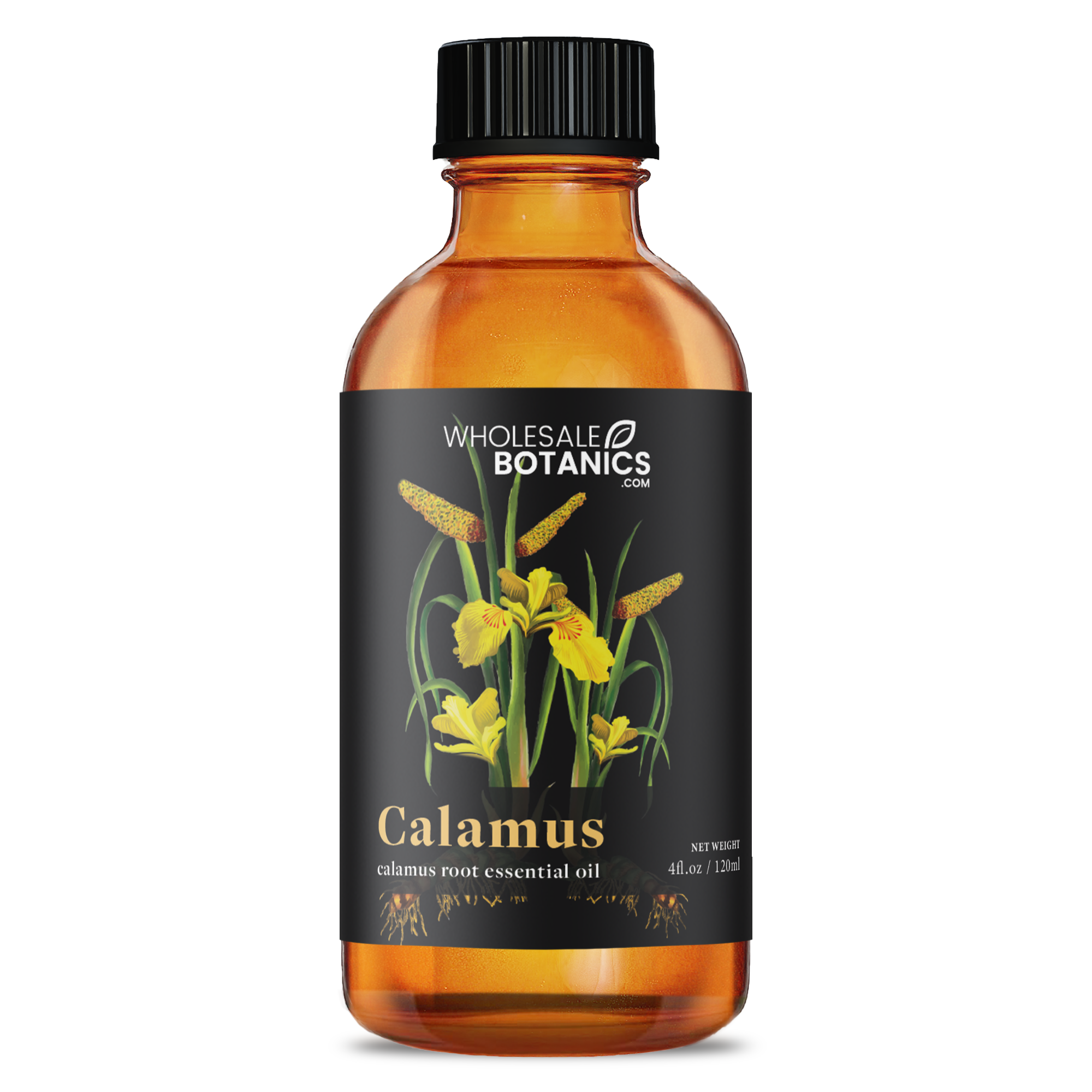The image features a professionally taken product shot of a small, 120 milliliter (4 fluid ounces) amber bottle with a ridged black cap. The bottle is filled up to about an inch from the top and casts a slight shadow on a pure white background, typical for stock photos used in online stores like Amazon. The center of the bottle is adorned with a black label inscribed with "wholesalebotanics.com" in white lettering, accompanied by a leaf graphic next to the word "Wholesale." Prominently displayed in the middle of the label is a vivid image of a yellow iris, accompanied by several buds and greenery in the background. Below the iris, the label reads "Calamus" in bold yellow font, followed by "Calamus Root Essential Oil" in white font.